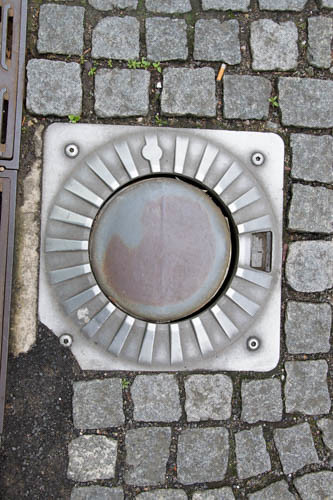In this overhead image, we observe a square metal plate embedded in a sidewalk comprised of neatly arranged, gray square stones. The metal plate functions as a light fixture and is secured with four screws. The bottom left corner of the plate has been chipped, revealing the dark, earthy ground beneath. The light fixture features a circular inner structure, part of which appears transparent. Within this circular structure lies another, smaller concentric circle, marked by a distinct pink spot. Additionally, lines extend from the edge of the outer circle towards the innermost part. On the metal plate, a discarded cigarette butt and tiny leaves are visible, adding to the scene's detail.